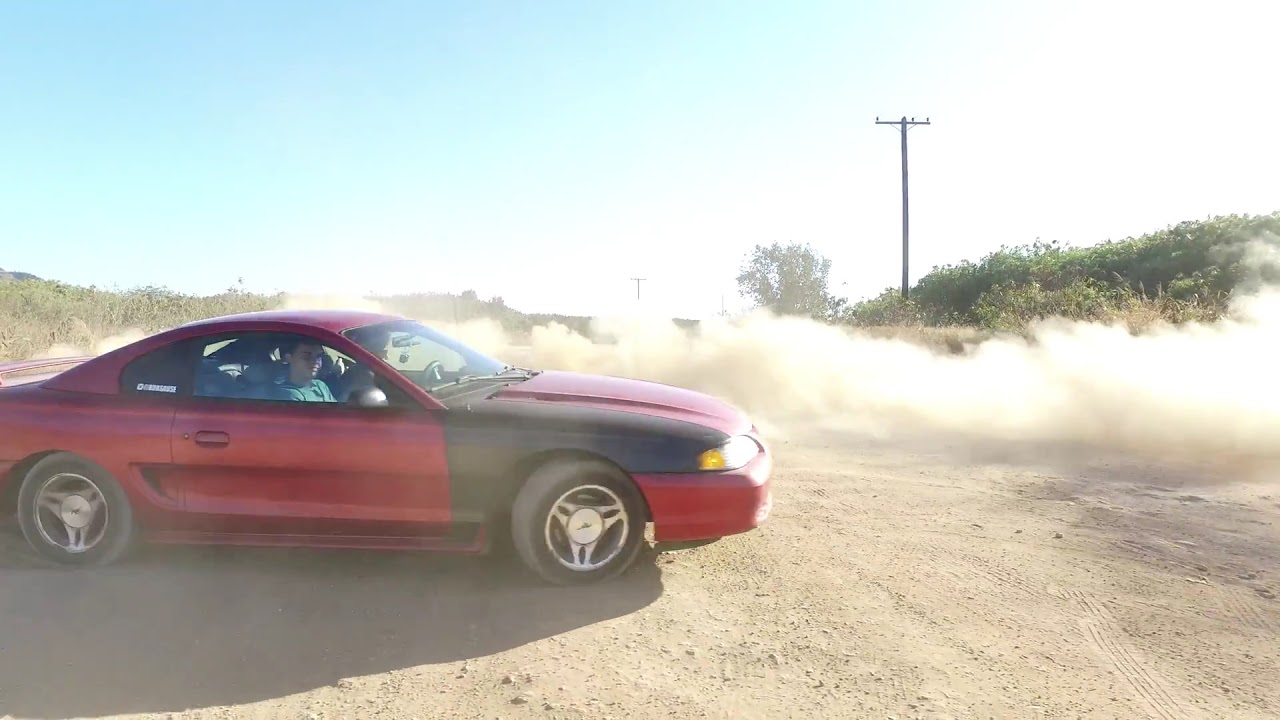The image features a vibrant, red sports car positioned center-left on a dusty dirt countryside road. The car, adorned with a black fender above the right front tire, is a two-door vehicle with no back door. Inside the car, there are two young males; the one in the passenger seat is wearing a blue shirt, while the driver, in the foreground, sports a black shirt. The scene is set under a cloudless, light blue sky. Various tire tracks crisscross the road, and a prominent cloud of dust rises, likely kicked up by the car speeding from right to left. To the right side of the image, the road slopes up into a small hill covered with green vegetation. In the distance, a tree stands tall alongside some power lines, adding depth to the rustic backdrop.